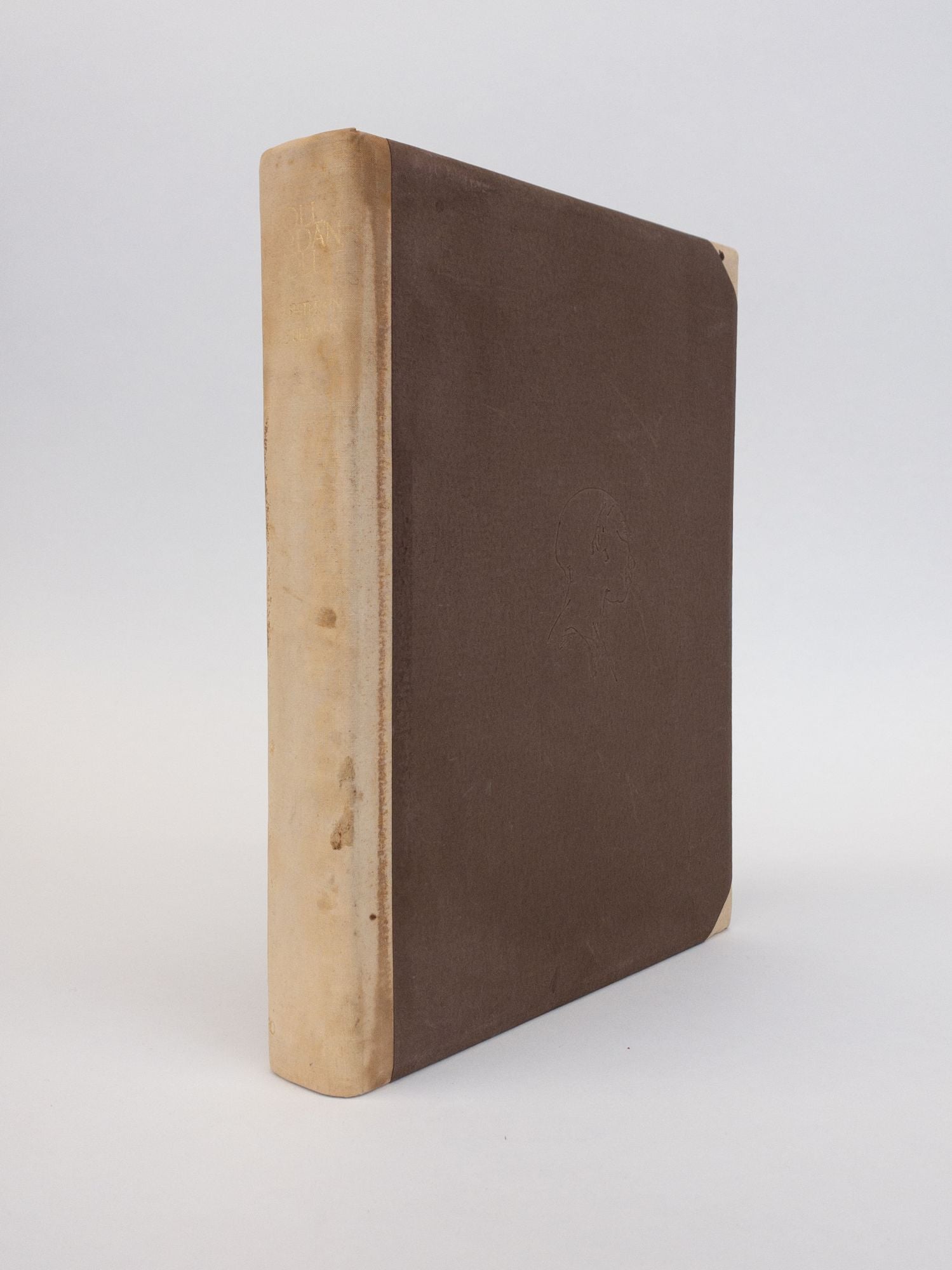The image features a rectangular object, likely a book, positioned upright with its front oriented towards the southeast and the side towards the southwest. The background is a clean, white space with soft, professional lighting emphasizing its features—indicative of a product photograph. The book's spine appears to be a worn, white leather color with barely legible, faded text near the top. The front cover is a medium-tone brown with a dark brown top, and the right side hosts light brown triangular segments at the upper and lower corners. The height of the book is greater than its width, giving it an elongated appearance. The depth of the object, visible from the side, is narrow, measuring about 1 to 2 inches. The white background and the meticulously draped textured paper suggest a meticulously staged environment designed to highlight the book’s intricate details, which includes subtle stains and what might be a profile of a face on the cover.